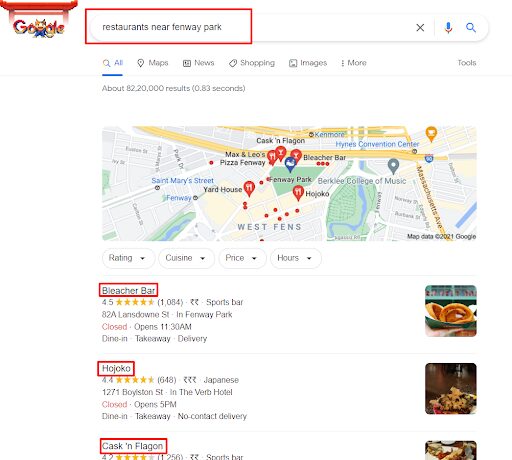The image depicts a Google search results page, likely performed around the time of Chinese New Year, as indicated by the festive, Asian-themed Google logo. The search query "restaurants near Sunway Park" is prominently displayed at the top. The results yield approximately 822,000 entries in just 0.83 seconds. Highlighted restaurant listings include Bleacher Bar, Hojoko, and Cask 'n Flagon, complemented by a map on the right side pinpointing their locations around Sunway Park. Notably, the presence of a rupee symbol suggests the search may have been conducted via a localized version of Google for India. Despite the currency hint, the search context is inferred to be in Boston.